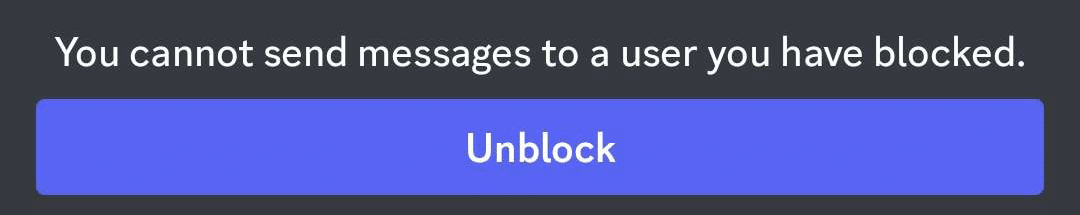The image depicts a notification, likely from the Discord application, indicating that the user cannot send messages to someone they have blocked. The notification is presented within a black rectangular box, featuring white text that states, "You cannot send messages to a user you have blocked." Below this message is a prominent rectangular "Unblock" button, which spans the entire width of the notification and is colored in a blue or purple hue consistent with Discord's color scheme. The design and color palette strongly suggest that this notification belongs to Discord, although it is noted that similar features could theoretically appear in other messaging services like Facebook Messenger.